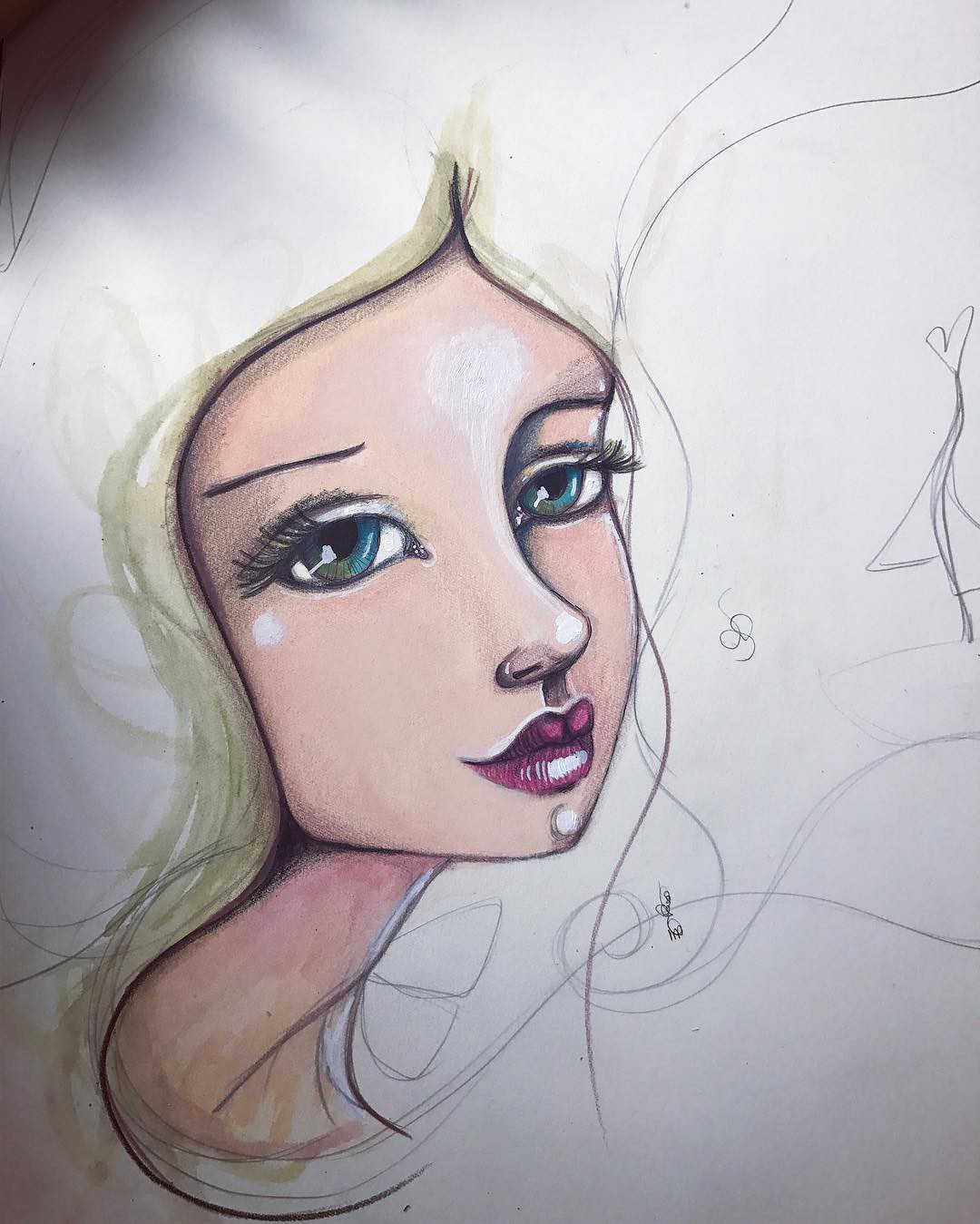This artwork features a close-up, three-quarter view of a female face, distinctly sketched and partially colored on a white piece of paper. The subject, an animated woman, has striking greenish-bluish eyes that are highly detailed, with visible highlights enhancing their depth. Her face and neck exhibit natural flesh tones subtly blended with hints of pink and red, possibly created using watercolor or colored pencils. Her neck is notably abstract, twisting slightly at the base, breaking from realistic proportions. The lips are full and vividly red, accented with white highlights, while her eyebrows and elaborate dark eyelashes contrast sharply against her mostly outlined facial features. The hair is only partially colored, with soft blonde tones outlining her head and extending below her neck. The image is artsy and abstract in its execution, capturing the essence of the subject with selective detailing. Notably, the artist's signature is inscribed in small, hard-to-read letters, adding a personal touch to the composition.